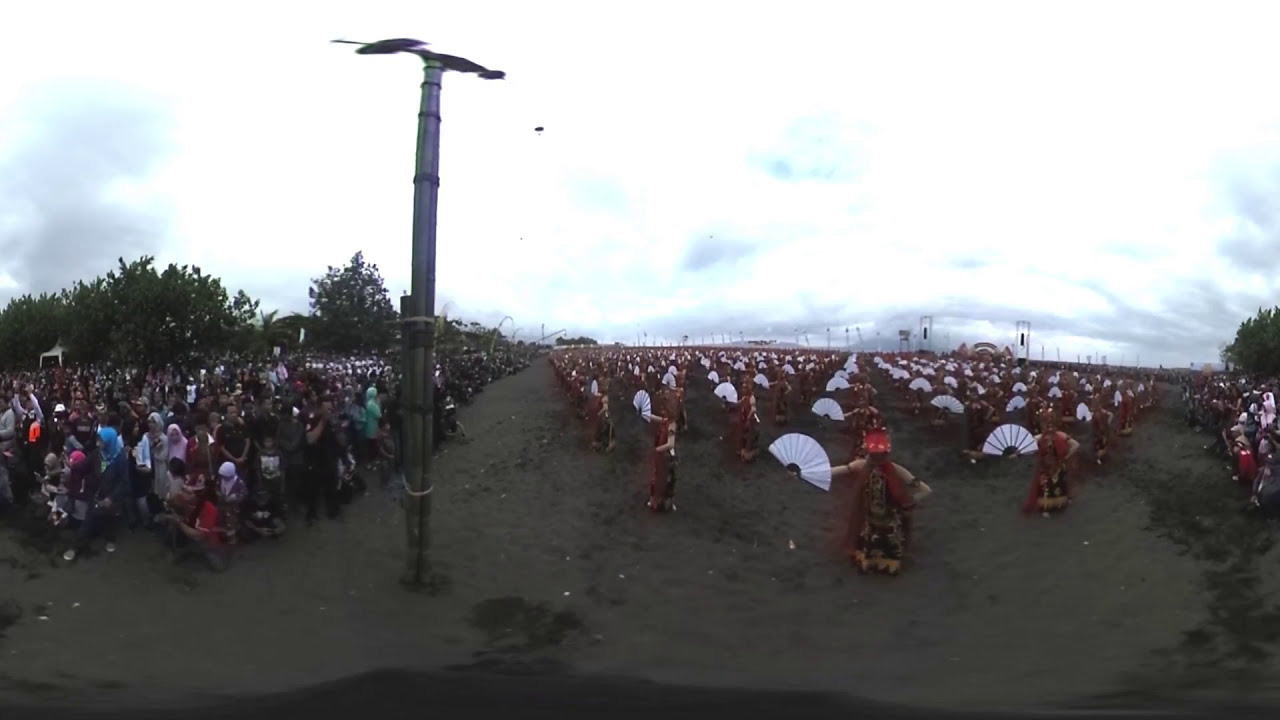In this photograph, taken on a cloudy day with a silvery sky, the scene appears to be a vibrant outdoor festival or ceremony, possibly in Japan, characterized by intricate cultural displays. The ground is a dark, earthen tone, and slightly left of center stands a tall pole, potentially a light pole. To the left of the pole, a dense crowd of spectators of varying ages and dressed in colorful attire gather in front of a row of low trees. On the right side, there are numerous rows of performers, dressed in traditional Asian, likely Japanese, costumes that extend to the ground and appear sleeveless. These costumes predominantly feature red, with accents of black and gold. Each performer holds an open white fan and wears a reddish hat. To the far right, another group of spectators watches the event as it stretches far into the horizon.